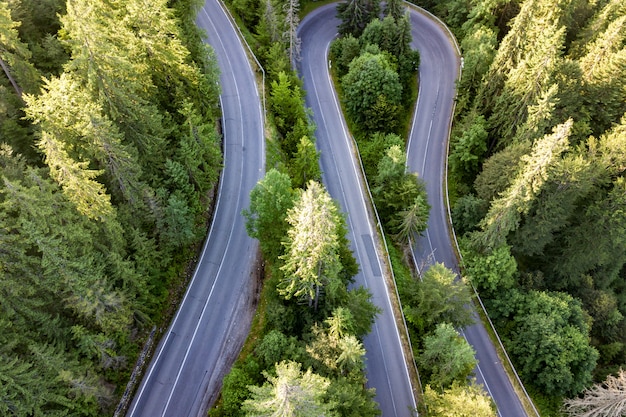This horizontal aerial photograph captures a densely forested area with mature, tall pine trees, bathed in bright, mid-day sunlight, suggesting it is taken during summer. Dominating the scene is a winding, paved road that starts from the top left and meanders downwards, curving to make a notable U-turn before continuing its serpentine path. The dark pavement is clearly marked with a white line down the middle and two white lines on either side. No vehicles are apparent on this road. The dense canopy of trees covers both sides of the road and extends between the roads, creating a lush, green corridor through which this roadway twists and turns.